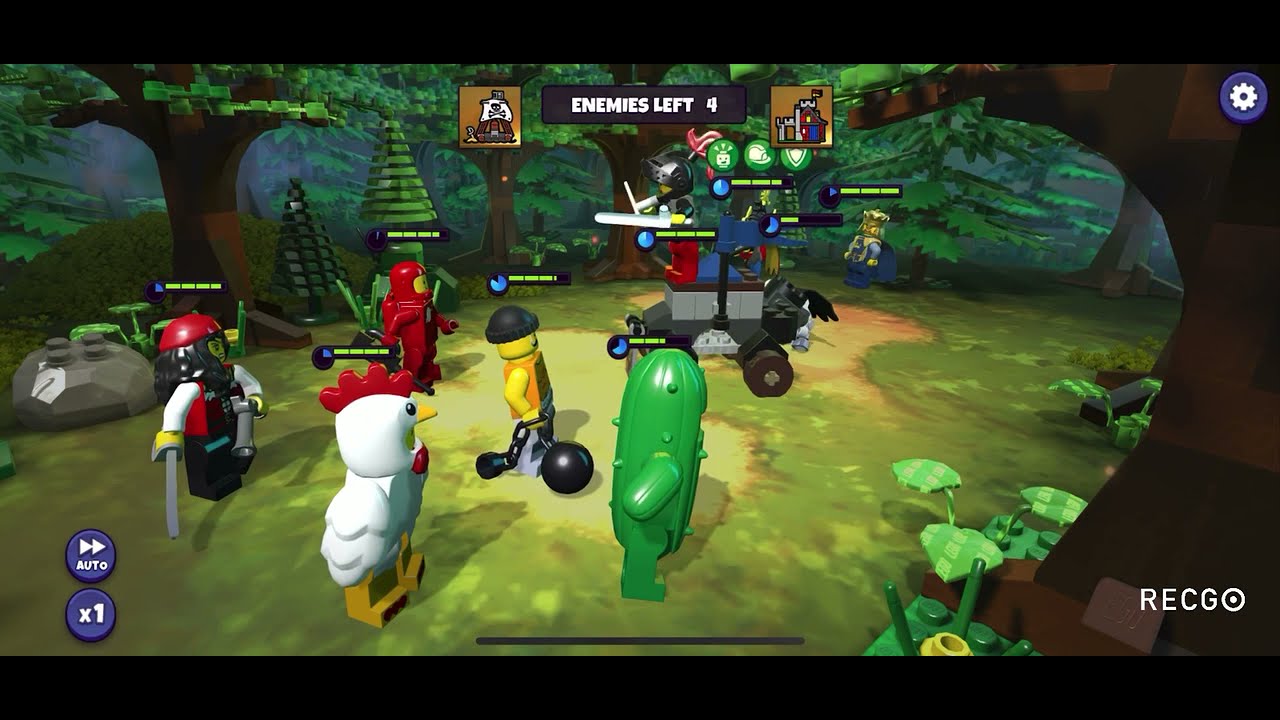The screenshot depicts an animated, cartoony scene from a video game, resembling a Lego-themed environment. The setting is a forest clearing surrounded by tall green trees and lush green grass, brightly lit compared to the darker woods around it. In the center, various distinct characters, reminiscent of Lego figures, are seen collaborating on constructing or maneuvering a contraption on wheels. The characters include a green cactus, a yellow figure with a black hat standing next to a black ball, a person in a white chicken suit, a character in a red space suit, a pirate-like figure, and a man dressed in blue standing behind the contraption. Another character, possibly dressed in all black, appears to be driving the contraption. The scene includes heads-up display elements, with text reading "enemies left: four" flanked by two icons near the top and a gear symbol in the upper right corner. Additional UI buttons labeled "auto" and "x1" are visible in the lower left, enhancing the gaming interface. Overall, the game scene is a vibrant and engaging forest enclave bustling with colorful Lego characters.